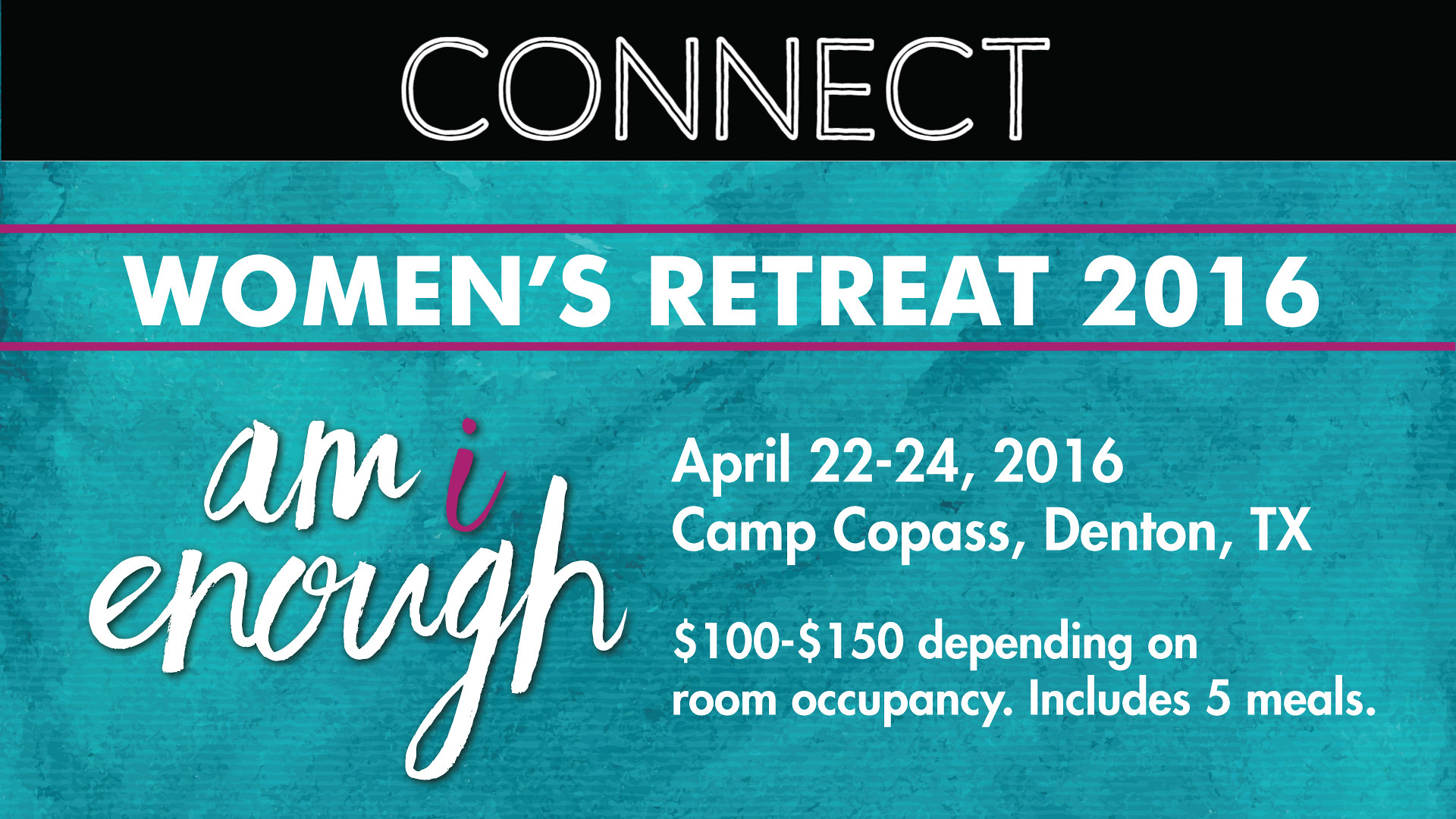This is an advertisement for the Women's Retreat 2016, featuring a sleek and striking design. At the very top, a black color block showcases the word "Connect" in a white outline font, black in the center. Below, on a textured blue, almost tie-dye background, the text "Women's Retreat 2016" appears in bold white letters, bordered by two magenta horizontal lines above and below. To the left, a handwritten cursive font spells "Am I enough?" in white, with the "I" highlighted in magenta. On the right, the event details are listed in white text: "April 22nd to 24th, 2016, Camp Copas, Denton, Texas". It mentions the cost, "$100 to $150 depending on room occupancy," and includes five meals.